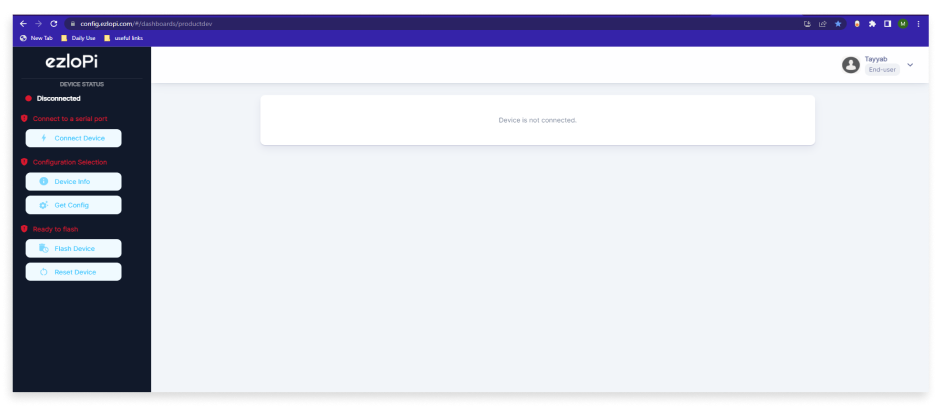This image, sourced from the website ezlopi, displays a somewhat blurry screenshot of a web-based interface. At the top, there is a prominent navigation bar with the URL "config.ezlopi.com/#/dashboard/product-dev" visible. The interface includes a white left arrow, a grayed-out right arrow, and a white refresh button for navigation and reload functionality.

Below the navigation bar, there is a tab section featuring options such as a new tab button, "Daily Use" option, and "Useful Links." On this section, there is also an indicator labeled "Device Status: Disconnected."

Additionally, users have the option to connect to a serial port via a "Connect Device" button. The interface also provides various configuration tools including a "Configuration Selection," a "Device Info" button, a "Get Config" button, and an expanded option labeled "Ready to Flash." For device management, there are two primary action buttons: "Flash Device" and "Reset Device."

The 
layout and annotations suggest an interface intended for device configuration and management, though the blurry quality of the image may obscure finer details.